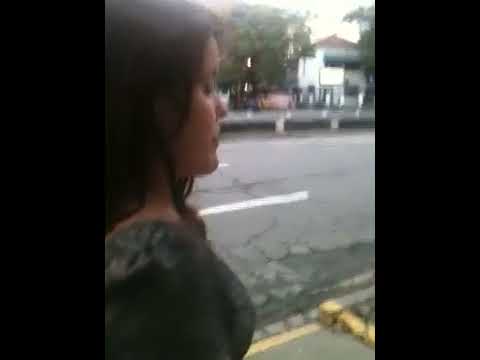The image portrays a side view of a woman walking on a cracked, gray sidewalk or paving made of asphalt and concrete. She has long, dark brown hair that falls over her shoulders and appears to be in her mid to late twenties. She is wearing a top that seems to be either light green or gray, and her eyes appear to be closed or looking down. The photo is slightly blurred and pixelated, capturing just the top half of her shoulder and the side of her face. The background features a large green-leaved tree and another tree, both flanking a white residential building with a brown or orange roof. A guardrail or barrier runs along the road, which has white traffic markers and looks rutted and cracked. The scene is set during the daytime, under a sky that appears white in the image. The left side of the image includes the woman’s silhouette, while the right side showcases the walkway, road, and background elements, including yellow markings and side roadblocks.